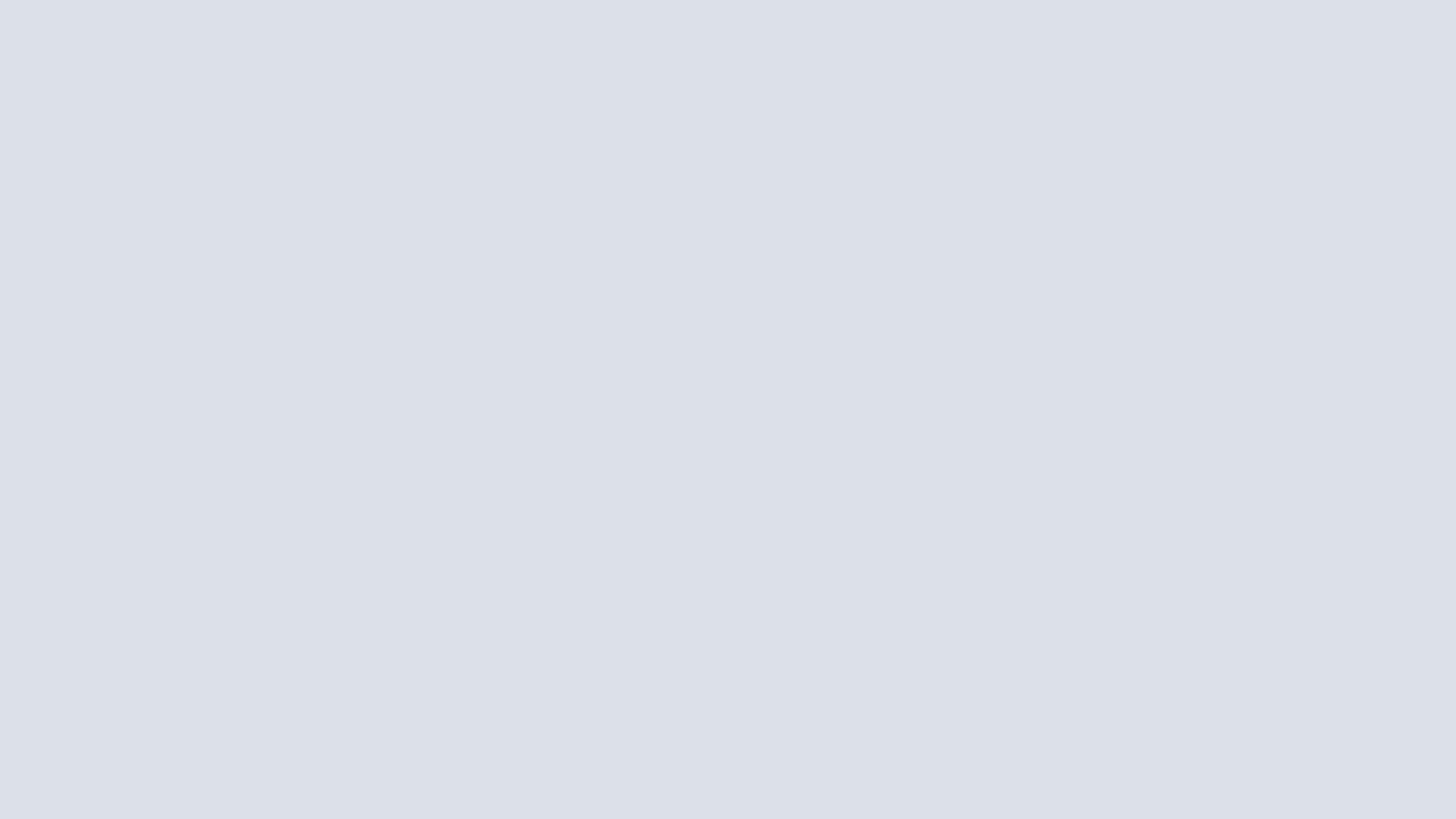This image features a medium gray rectangle with slightly longer top and bottom sides compared to the left and right sides. The gray hue has a subtle, swirling mixture with white, giving the base color a somewhat varied texture. The rectangle has no border and is set against a plain white background. It contains no additional elements, such as pictures, text, or advertising. The image is a plain gray box, offering no contextual information or explanatory content.